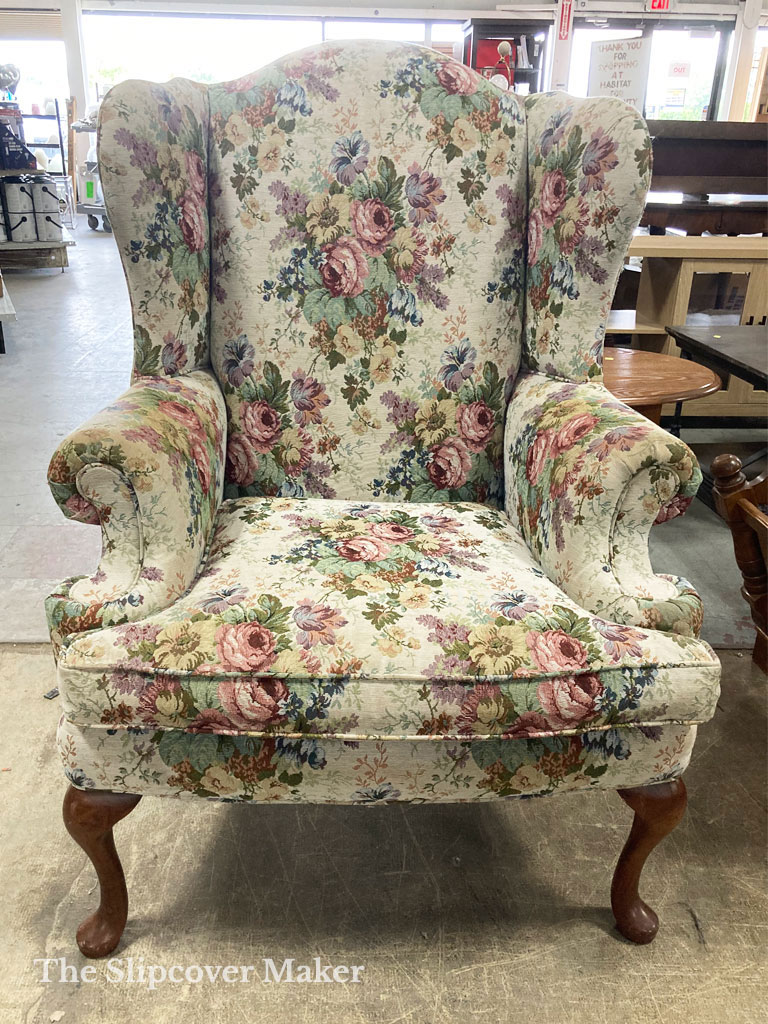This vertically oriented photograph features an old-style wingback armchair prominently placed in the center. The chair's upholstery is a cream or beige color adorned with a detailed floral pattern that includes pink roses and green leaves, giving it a distinctly nostalgic aesthetic. Additionally, there are hints of red and yellow flowers interspersed in the design, enhancing its rich, floral appearance. The armchair has padded armrests and rests on short, dark brown wooden legs shaped like feet.

Situated on a scratched tile floor, the chair appears to be in a mixed-use space, possibly an office setting merging into a warehouse or loading dock, evident from the visible large window with light shining through, a door topped with an exit sign, and furniture including a round brown table and a shelf behind it. The lower left corner of the image features the text "The Slipcover Maker," indicating this might be an advertisement showcasing the chair's reupholstered look.